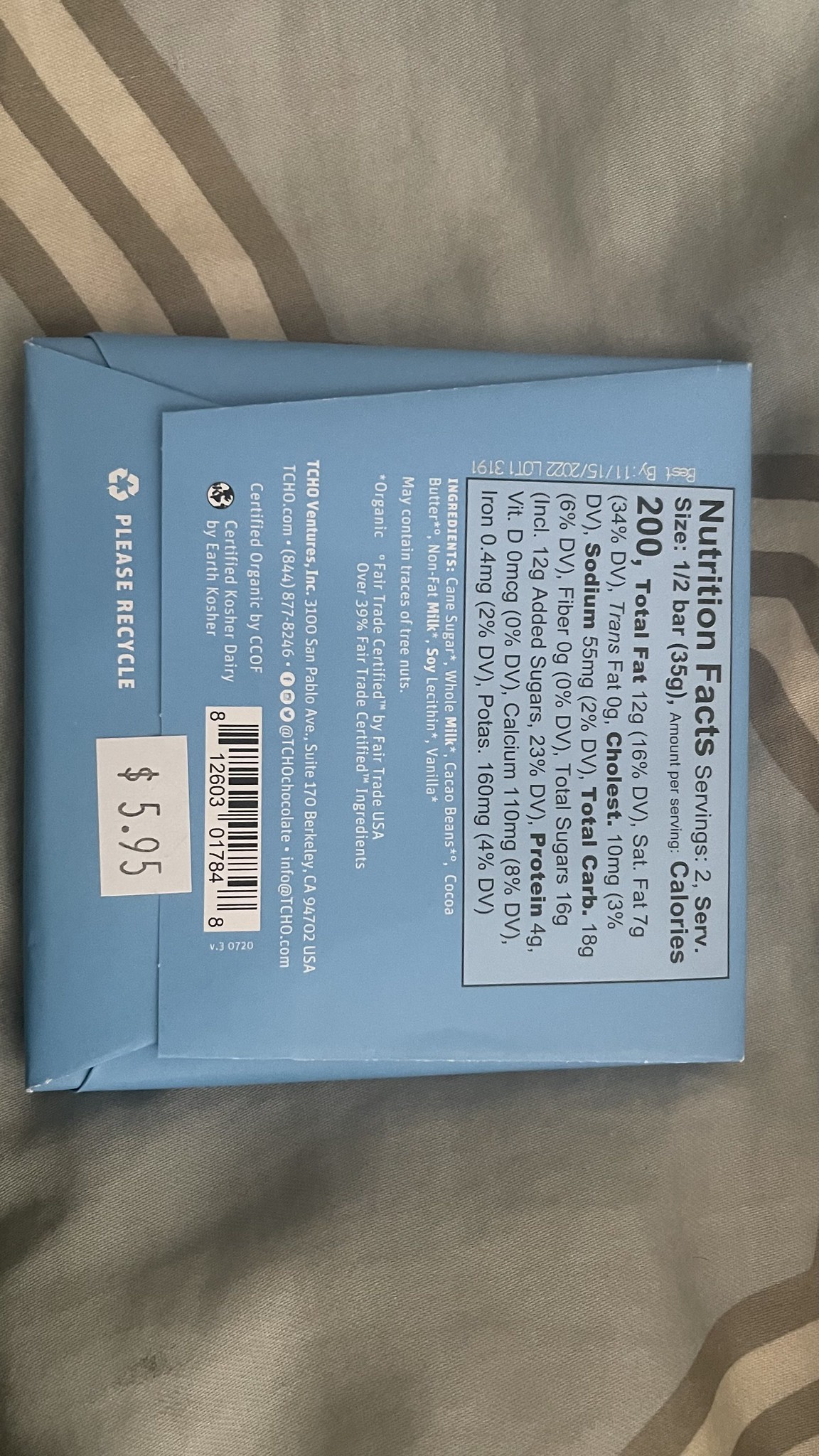This color snapshot, taken from a top-down angle, depicts a blue paperboard food container, possibly for nutritional bars or chocolate, that needs to be rotated 90 degrees to the left for easier reading. The container rests on a rumpled fabric background that is primarily khaki with a beige, brown, and white striped pattern. A small white sticker on the box displays a price of $5.95, and there is a symbol urging to "please recycle." The container features detailed nutrition facts and ingredient information in white, with black text within the nutrition facts rectangle. Specifics include two servings per container, 200 calories per serving, 4 grams of protein, and 0.4 milligrams of iron, although much of the text is too small to read clearly.